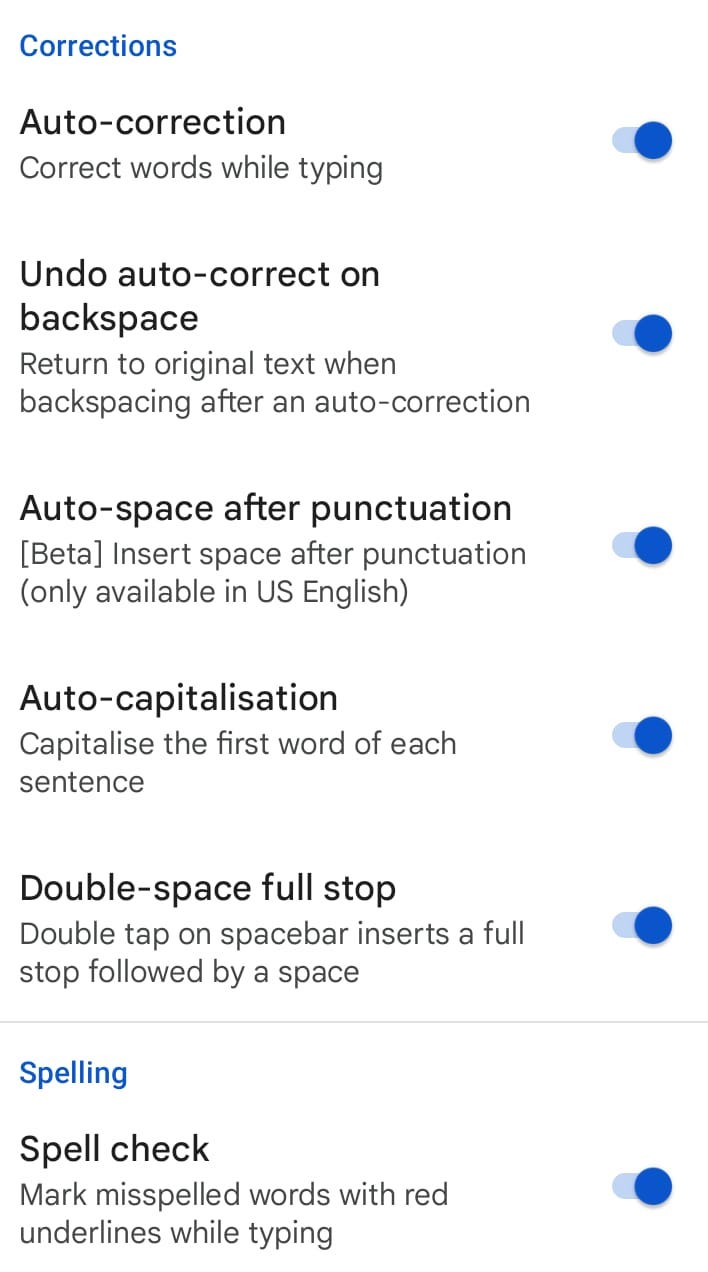This is a cropped mobile screenshot displaying the Corrections tab under the Settings menu, with a clean white background. At the top left corner, the word "Corrections" is prominently featured in bold blue font. Below, there's a comprehensive list of subcategories, each accompanied by a toggle switch positioned to the right.

The first subcategory, titled "Auto Correction" in bold black font, includes an explanatory note underneath: "Correct words while typing" in small grey letters. The corresponding toggle switch, situated to the right, is activated and highlighted in blue.

The next subcategory is "Undo Auto Correct on Backspace", which also has its toggle switch turned on. This is followed by "Auto Space After Punctuation," "Auto Capitalization," and "Double Space Full Stop," each with their respective toggle switches activated.

Beneath these, lies the "Spelling" category, featuring a sub-option titled "Spell Check" with an enabled toggle switch. Evidently, all toggle switches under the Corrections section are set to "On".

*Thank you for viewing.*